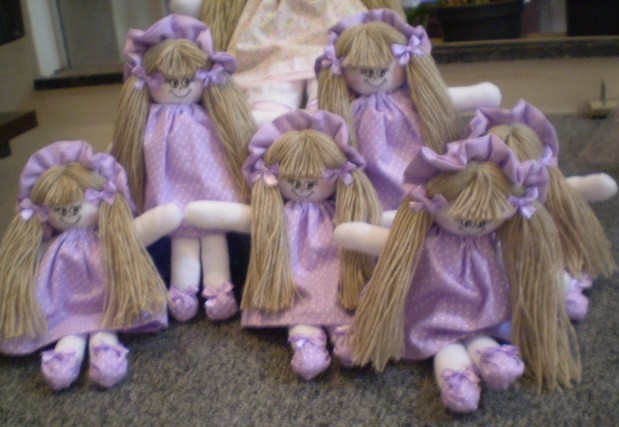In this image, there are six identical rag dolls arranged in a row on what appears to be a dark gray and tan carpet. Each doll has straw-colored hair made of yarn, styled into long pigtails adorned with blue ribbons and small blue bonnets. Their faces feature painted-on eyes and a smile, giving them a cheerful appearance. Each doll is dressed in a blue dress with tiny bows and blue slippers, accentuating their uniform look. The dolls appear to be leaning on each other. Behind them, there's a larger doll that seems to share the same straw-colored hair and facial features, suggesting it's a bigger version of the same type of doll. The larger doll, however, appears to be dressed differently, in a white dress, contrasting with the blue outfits of the six smaller dolls. The scene portrays a neatly arranged collection of factory-produced dolls, captured in what looks like a cozy indoor setting.